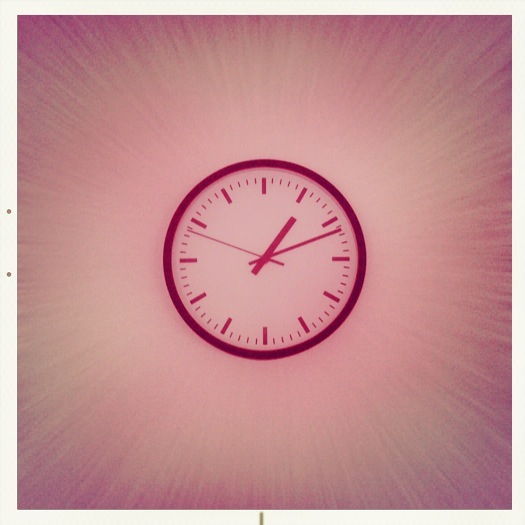The image depicts a vibrant pop art-style illustration of a clock, characterized by a dynamic and colorful composition. A clean white border frames the artwork, which showcases a striking background gradient transitioning from a darker pink on the periphery to a dull white-yellow shade at the center. The overall effect resembles an explosion or speed lines radiating outward from the center, enhancing the visual impact.

Central to the image is a prominent black analog clock, occupying approximately 30% of the canvas. The clock features a minimalist design with the numerals represented by straight lines, requiring familiarity with traditional clock face positions to decipher the time. Encased in a sleek black circular trim, the clock hands indicate the time as just past 1:10, with the minute hand pointing slightly past the 10 and the hour hand near the 1. The second hand is poised almost towards the 10, adding a subtle sense of movement to the piece. This detailed and vibrant depiction merges the bold aesthetics of pop art with the functional design of an analog timepiece.